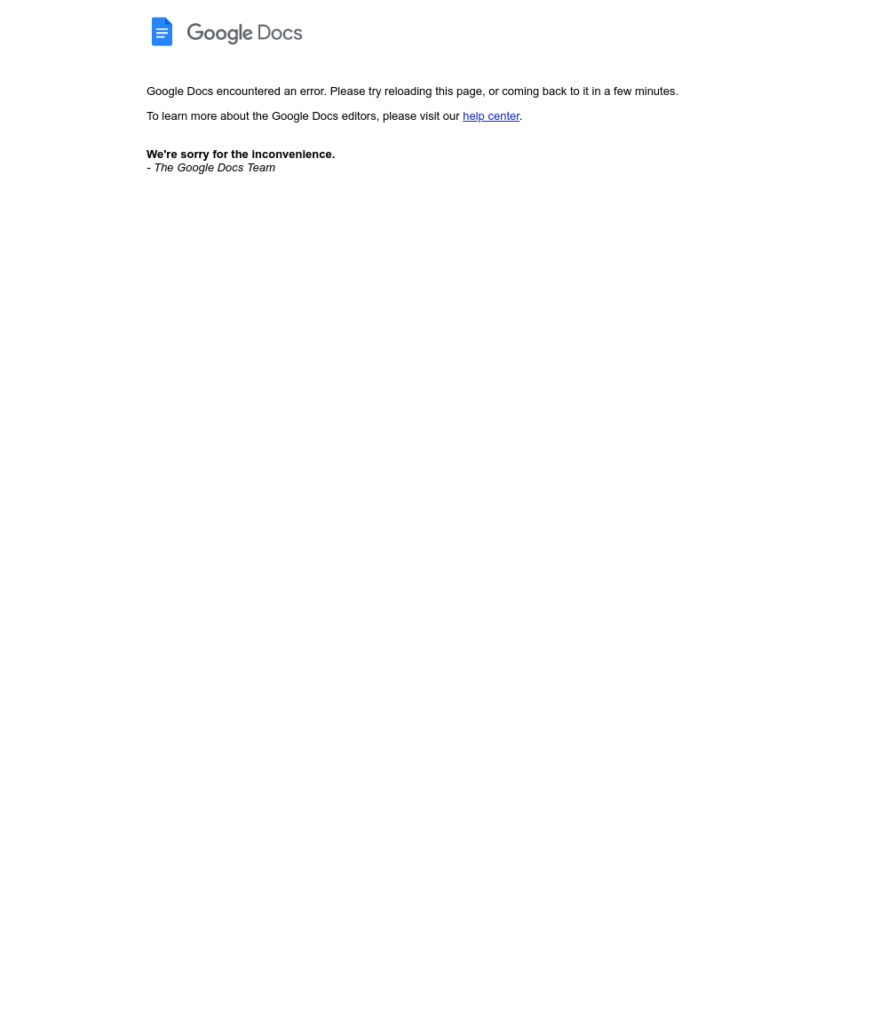The image displays a Google Docs error message against a plain white background. Prominently featured at the top is the Google Docs logo, with "Google" in bold gray font and "Docs" in a lighter gray font. To the left of the text is a blue icon resembling a piece of paper with its upper-right corner slightly cut off, containing three horizontal white lines.

Beneath the logo, in small gray font, the message reads: "Google Docs encountered an error. Please try reloading this page, or come back to it in a few minutes." 

On the next line, the message continues, "To learn more about the Google Docs editors, please visit our Help Center," with "Help Center" highlighted in blue and underlined, indicating a hyperlink.

Following a slightly larger space, there is a bold statement in black font: "We're sorry for the inconvenience." 

Directly below this, in italicized gray font, it reads: "– The Google Docs Team," with each word capitalized.

The remaining portion of the image comprises extensive white space, ending near where a recording button would typically be situated, though no additional elements or text are visible.